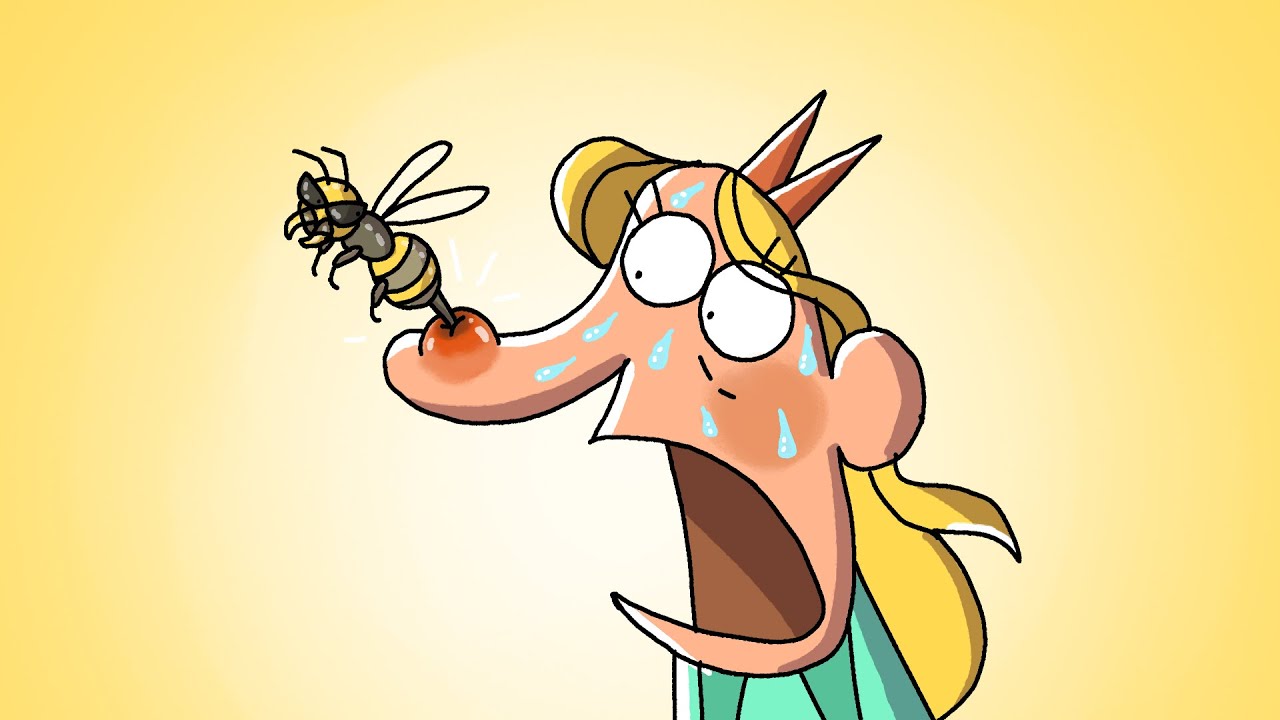The image depicts a cartoon character being stung on the nose by a bee. The background features a radial gradient transitioning from white at the center to light yellow at the edges. The character, appearing to be a woman or potentially a man, is looking to the left with an expression of shock, mouth wide open, and teardrops or sweat droplets coming from the eyes and forehead. The character has long yellow, possibly golden, hair and is wearing a turquoise green shirt. Notably, there are two red, triangle-shaped accessories, likely ribbons or possibly small horns, on top of the character's head. The individual’s nose is drawn exaggeratedly long, protruding to the left, with a big red bump at the end where a bee, depicted with black and yellow stripes, white wings, and an anthropomorphic design that makes it appear to be wearing sunglasses, has its stinger stuck. This vivid and detailed cartoon captures the character's apparent distress vividly.